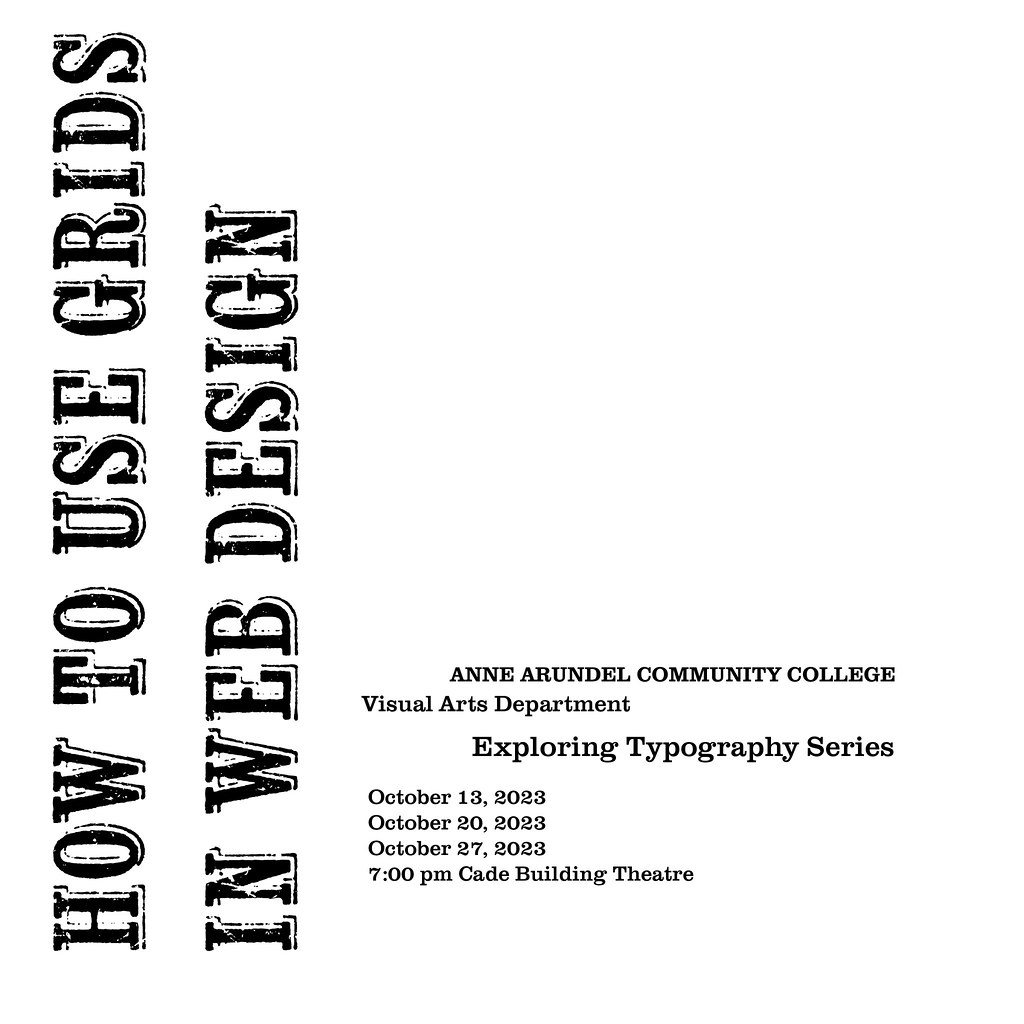The image depicts the title page of an educational book or presentation with a clean, white background. On the left-hand side, written horizontally in bold, black font with a shadow effect, are the capitalized words "HOW TO USE GRIDS IN WEB DESIGN," which require turning your head to read. Vertically aligned on the left, in smaller, normal print, is additional information: "Anne Arundel Community College, Visual Arts Department, Exploring Typography Series." Below this, the dates "October 13, 2023, October 20, 2023, October 27, 2023" are listed, along with the time "7 p.m." and the location "Cade Building Theatre." This collection of details suggests that the image announces a presentation series on the specified topic.